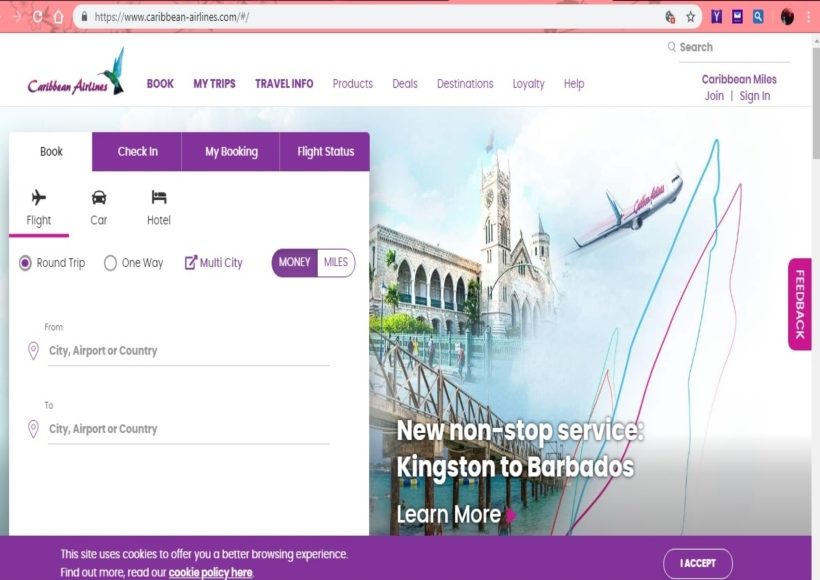The top section of the webpage displays a distinctive coral-colored bar labeled "Caribbean Airlines." Right next to the label is the airline's official website, featuring a captivating image of a hummingbird with its wings gracefully extended upward. 

The navigation menu offers various options, allowing users to explore tabs for booking flights, managing trips, accessing travel information, discovering products, finding deals, exploring destinations, joining loyalty programs, and seeking help. Above this menu, there is a search bar, along with links for viewing or joining the Caribbean Miles loyalty program.

The text across the site is embellished in a vibrant purple, contributing to the overall colorful aesthetic. Further down, there are visually appealing, artistically rendered images of various destinations Caribbean Airlines serves, accompanied by an illustration of a jet, symbolizing the airline's extensive reach.

A pop-up screen appears upon clicking the "Book" tab, which includes options for check-in, managing bookings, and checking flight status. The "Flight" section is selected, set for a round-trip, prompting users to input their departure and arrival locations. Travelers can choose to pay for their flights using either money or accumulated miles. However, in this particular instance, the specific locations of departure and destination have yet to be entered.